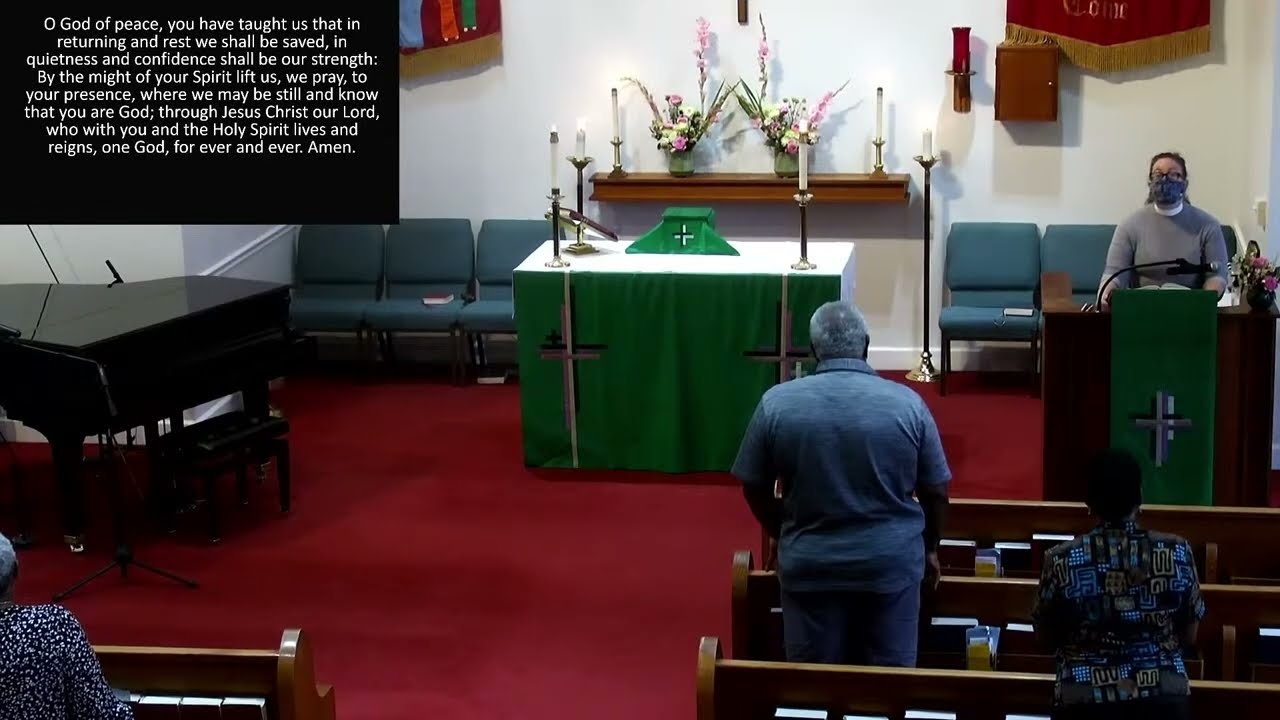The photograph captures the serene interior of a church setting. At the center of the image, pews are arranged neatly, with three individuals standing in them, engaged in attentive observation. A woman, likely the pastor, stands at a wooden lectern on the far right-hand side, donning a long gray sweatshirt, glasses, a white clerical collar, and a cloth mask. The deep brown wooden lectern is accentuated by a green cloth emblazoned with a white cross.

The altar, centrally located, is adorned with a green cloth featuring two white crosses, alongside candlesticks, adding to the sacred atmosphere. Behind the altar, blue chairs and various decorative elements such as flowers, candles, and shelves contribute to the room's solemn decor. A grand black piano is positioned in the far left-hand corner, creating a harmonious balance within the space.

Above the piano, prominently displayed in a black box with white text, is a prayer that reads: "O God of peace, you have taught us that in returning and rest, we shall be saved; in quietness and confidence shall be our strength. By the might of your Spirit, lift us, we pray, to your presence, where we may be still and know that you are God. Through Jesus Christ our Lord, who with you and the Holy Spirit lives and reigns, one God forever and ever. Amen." This encapsulates the reverent ambiance of the church.